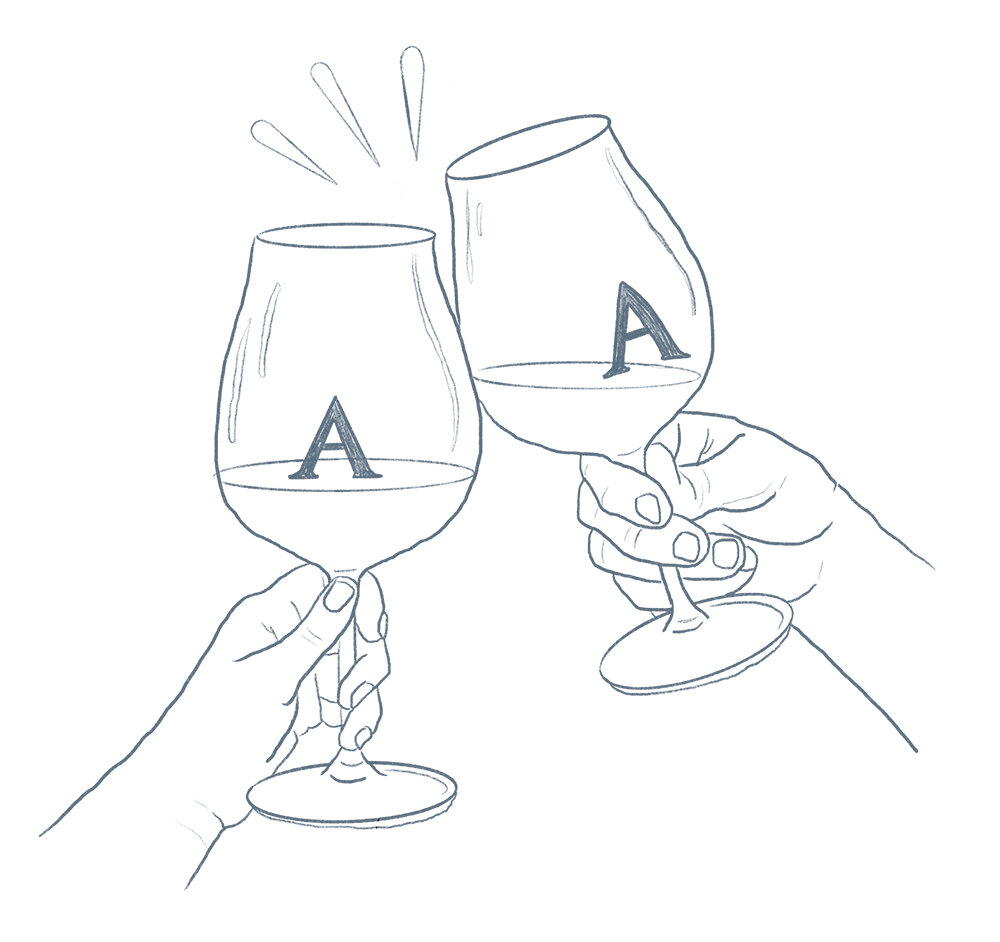This black and white ink drawing, set against a white background, depicts the scene of two hands toasting with wine glasses. The hands are each grasping the thin stems of the glasses; the left glass is held upright, while the right one is tilted at an angle. Both wine glasses, which feature a base, a thin stem, and a goblet-like cup, appear to be filled about halfway. Notably, each glass has the letters 'AA' printed on its surface, possibly indicating a reference to Alcoholics Anonymous. Above the clinking glasses, three teardrop-shaped marks suggest the sound or splash from the toast. The entire composition has the characteristic simplicity of a stencil or a minimalistic graphic, with all elements rendered solely in black ink against the plain white backdrop.